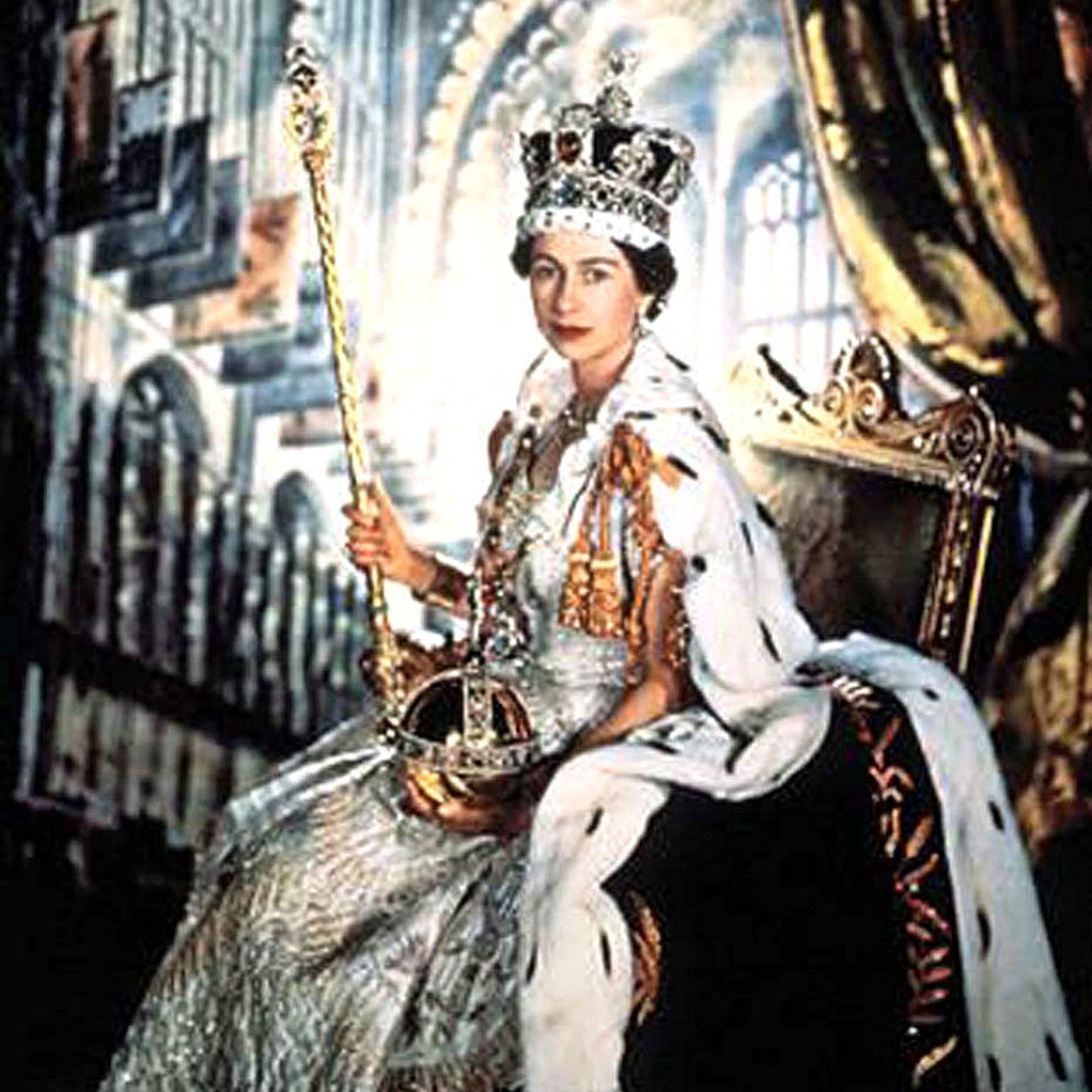This photograph features a young Queen Elizabeth seated on an ornate throne, surrounded by the luxurious interior of what appears to be a palace. Her dark brown hair is styled short, and she wears an elaborate crown adorned with jewels and a distinctive piece on the top. In her hands, she holds a gold scepter and another crown. Her attire is majestic: a silver and gold, intricately designed dress complemented by a white fur shawl cascading to the floor, complete with a fur collar. The regal outfit is further embellished by a beautiful blue velvet robe. She is adorned with makeup, including lipstick, and earrings. The backdrop includes sumptuous drapes and a large window that allows light to pour through, hinting at the grandeur of her surroundings. This image likely commemorates an important moment in her reign, capturing her in full royal regalia, looking directly toward the photographer.